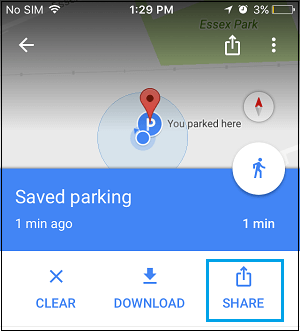Screenshot of Google Maps on a phone showing parking details. At the top left, the status bar indicates "No SIM" with Wi-Fi connected, and the signal strength is shown with three out of four bars filled. The time displayed is 1:29 PM. On the right side of the status bar, there's a clock icon indicating an alarm is set, and the battery level is critically low at 3%.

In the Google Maps app, the user has dropped a pin marking their parking spot with the label "You parked here." The pin has a timestamp noting "Safe parking one minute ago" in white font on a bright blue background. The map reveals that the user has walked a little past the parked location.

At the top of the map, "Essex Park" is visible, indicating the nearby area. The bottom of the screen features clearly outlined "Download" and "Share" buttons, with the "Share" button highlighted in blue. Additionally, there is an icon showing a walking figure, likely indicating a suggested walking route back to the parking spot. An arrow icon slightly below the top left corner suggests the option to exit the current view within the app.